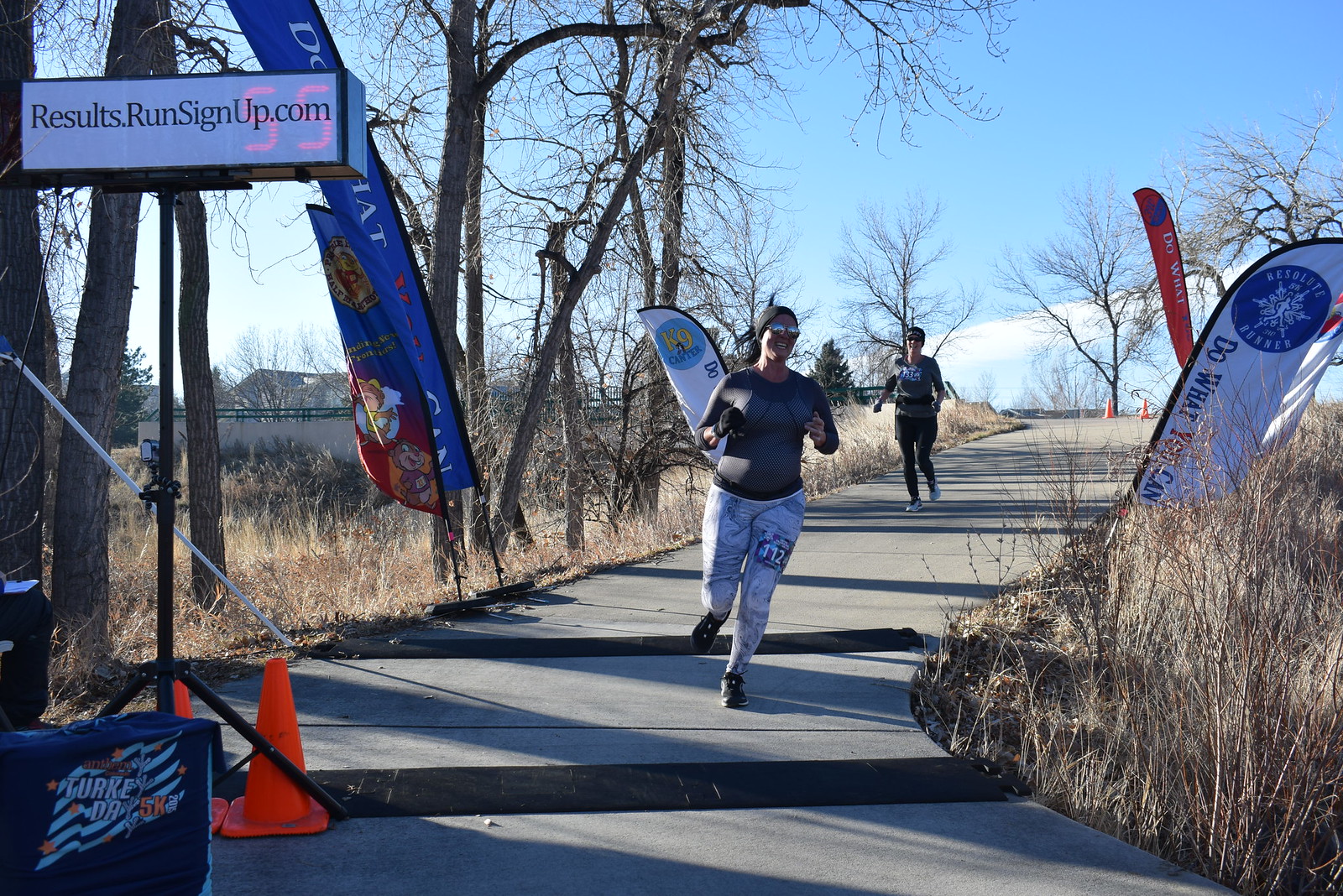The image captures an outdoor road race in the countryside during a sunny daytime. The central figure is a woman running down a paved gray asphalt road, wearing gray pants numbered 112 and a dark gray sweatshirt, along with gloves, sunglasses, and a knit cap. She is flanked by dry bushes and leafless trees. In the mid-background, another woman in dark attire is also running, with additional traffic cones scattered along the route. Prominent signs include a blue and white one with a snowflake saying, "do what you can," and a red one partially obscured with the same message. A sign in the lower left corner reads "resultsrunsignup.com" alongside the number 55. The sky above is a bright blue with white clouds. Shadows cast by the sun filtering through the bare trees add texture to the scene. A watermark featuring an American flag and "Turkey Day" is visible in the left-hand corner, highlighting the event's theme. Overall, the image is vibrant with a mix of colors including light blue, white, gray, brown, red, and orange, and vividly captures the energy and setting of the race.